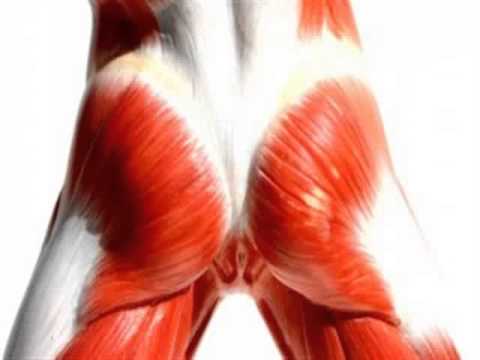The image is a highly detailed 3D rendering of the muscle structures beneath the skin of a human, specifically focusing on the area from the lower back down to the mid-thigh, viewed from the rear. The prominent feature is the musculature of the buttocks, depicted in vivid, stringy red muscle fibers. The background is white, reinforcing the medical illustration aesthetic often seen in textbooks or doctor's office posters. The image is interspersed with white sections along the outer thighs, lower back, and beneath the buttocks, possibly representing ligaments or connective tissue. The red muscle striations also appear on the inner thighs and the sides of the lower abdomen. A dark area is present in the middle of the lower back, flanked by white sections. The legs are slightly apart, and intricate ridges highlight the anatomical details. The overall impression is one of a precise educational tool designed to illustrate the muscular anatomy from the lower back to the upper thighs.